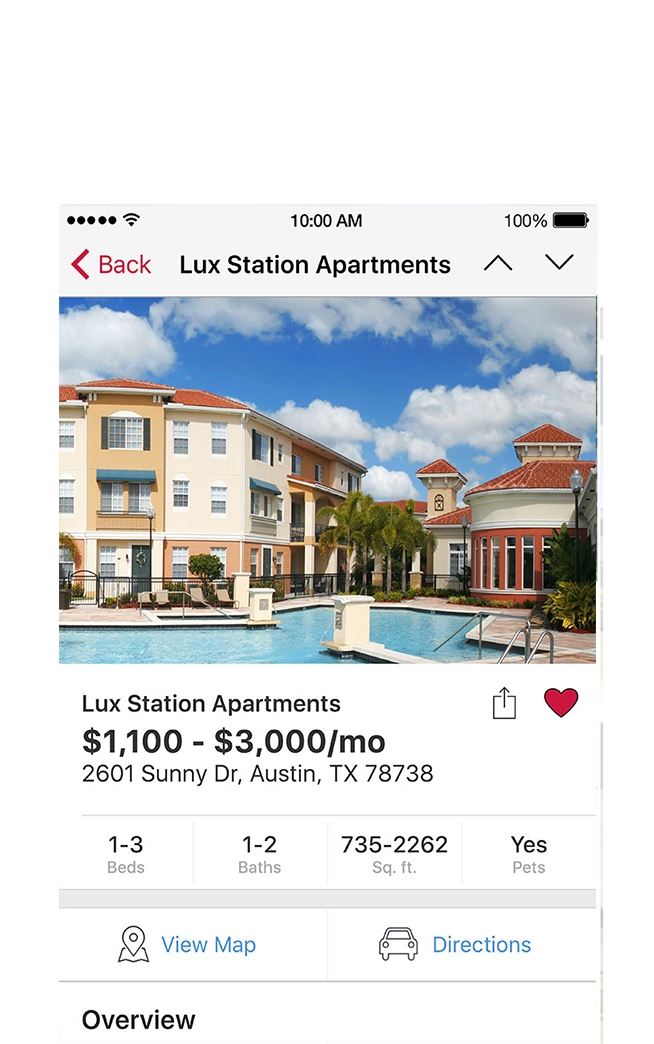The screenshot displays a mobile interface from an app or website dedicated to apartment listings. The device shows it is currently 10 a.m., with full Wi-Fi signal and 100% battery life indicated at the top of the screen. 

At the top left of the interface, multiple dots, likely representing a menu or navigation indicator, are present with a small Wi-Fi icon just beside them. 

Prominently in the center of the screen is the heading "Lux Station Apartments" in black text, with a red back button featuring a leftward arrow located just below the battery indicator on the right-hand side.

Below this heading is a photo of the apartment complex, which includes visible buildings and a pool. Accompanying the image are details about the apartments:
- Name: Lux Station Apartments
- Price Range: $1,100 to $3,000 per month
- Address: 2601 Sunny Drive, Austin, Texas 78738
- Bedrooms: 1 to 3
- Bathrooms: 1 to 2
- Square Footage: 735 to 2,262 sq ft
- Pets: Allowed 

Underneath the listing details, there are two buttons for interaction: "View Map" and "Directions." Also, at the bottom right corner of the photograph, a heart icon is displayed to indicate the option to favorite the listing, and it is currently filled in red, suggesting that it has already been marked as a favorite.